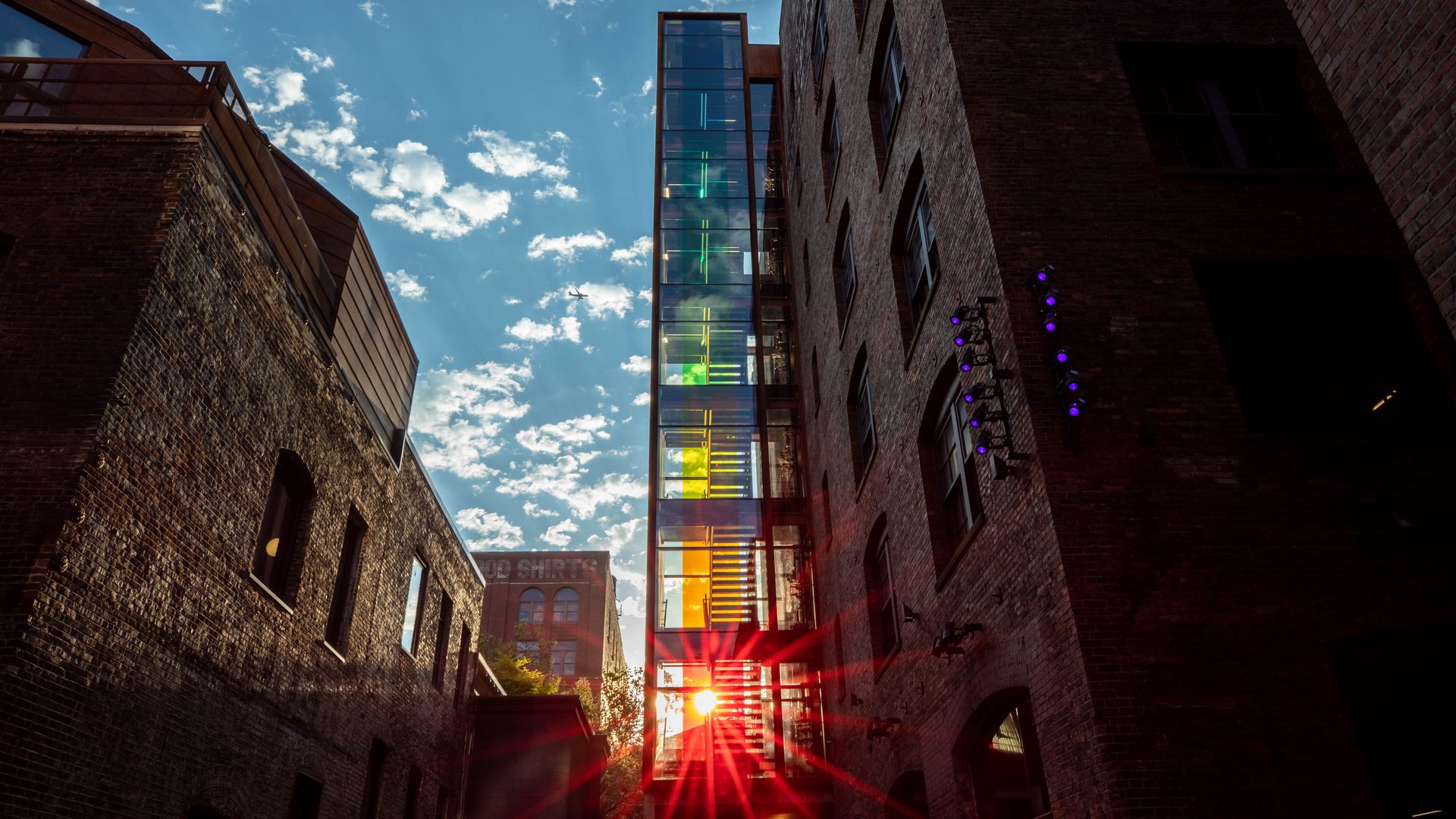In this detailed and vibrant urban photograph taken on a bright day, we observe an alleyway nestled between multiple stone and brick buildings, showcasing an intriguing cityscape likely situated in a gentrified city center. Dominating the scene is a six-story building with a striking glass-covered staircase running up its facade. The staircase is mesmerizingly illuminated in a spectrum of rainbow colors—from red at the bottom, through orange, yellow, green, and blue—captured vividly as the sun's rays hit the structure. The sunlight creates a captivating play of colors that adds a magical quality to the urban environment.

On the far left of the photograph, there's another stone and brick building with several windows, one of which is either lit from within or reflecting the sunlight, adding to the bright and airy feel of the image. In the background, a building with "shirts" prominently displayed at the top and large glass windows suggests a contemporary use, possibly as flats, hotels, or a museum.

Above, a clear blue sky adorned with speckled white clouds stretches across the horizon, adding depth and contrast to the scene. An airplane is seen flying far in the sky, contributing to the dynamic and lively atmosphere of this urban setting. At ground level, trees peek into the frame, adding a touch of nature to this urban photograph. The overall composition beautifully captures the essence of a vibrant city at daybreak.